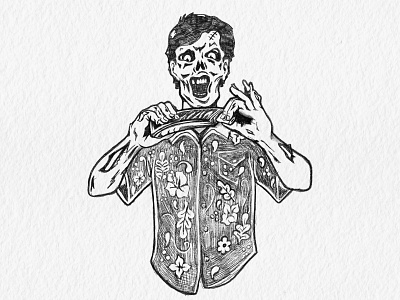This is an artwork depicting a detailed, black and white ink drawing of a male zombie centered in the image. The background is a light gray, which contrasts with the textured, watercolor-like paper that the drawing is on. The zombie's face is grotesquely distorted; his mouth is open in a classic zombie style, revealing the absence of his nose, with only the holes remaining. His face and forearms are marred with numerous gashes, one major wound on each arm, suggesting a brutal encounter. He has short, wavy dark hair. The zombie is wearing a Hawaiian shirt adorned with detailed hibiscus flowers and leaves, with a pocket on the upper left side. He is holding a rectangular object, which appears to be a sheath, and seems to be in the process of pulling something from it. This detailed and textured artwork evokes a scene reminiscent of horror films, with the zombie staring directly at the viewer, adding to its unsettling effect.